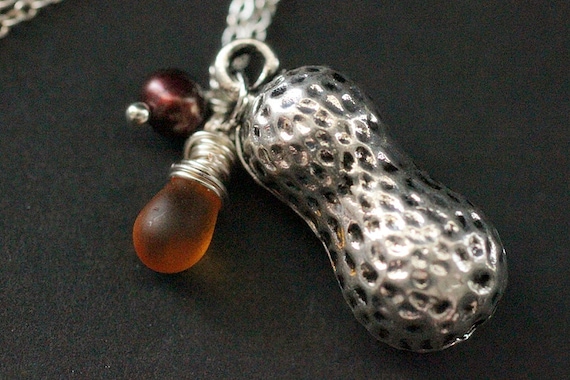In the foreground of the image, there is a detailed close-up of a silver charm shaped like a peanut, with dimpled surface mimicking the texture of a real peanut shell. This charm is attached to a small hook linking it to other jewelry that is just barely visible. Adjacent to the peanut charm, on the left side of the photograph, is another charm adorned with a wrapped silver wire and featuring a dark amber, teardrop-shaped bead that is almost translucent. Above this amber charm is a smaller, out-of-focus burgundy-colored bead. The backdrop of the image is a very dark gray, almost black, slate-like surface, which enhances the prominence of the highlighted charms.